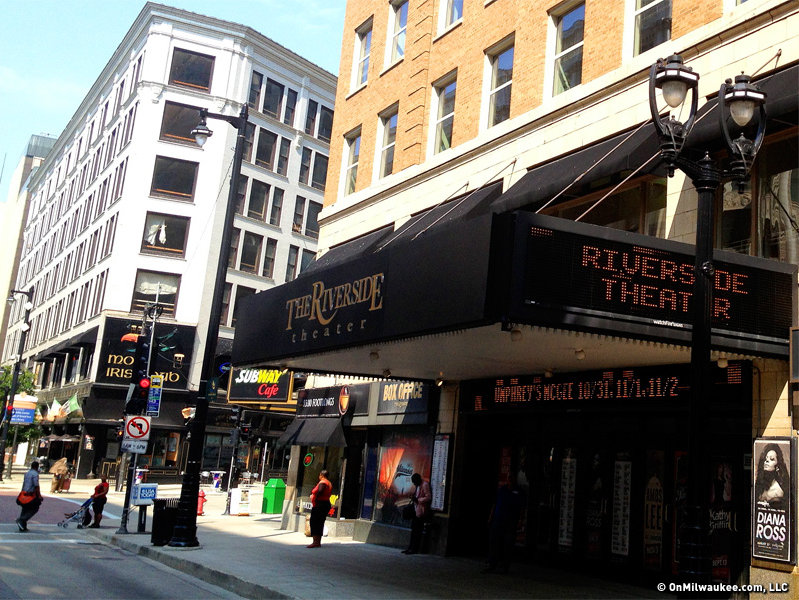The image depicts a bustling downtown city street, most likely in Milwaukee, with a vibrant urban atmosphere. Centered prominently in the scene is the Riverside Theater, easily identified by its distinctive black awning and gold-lettered sign that reads "Riverside Theater." An LED display above the theater's entryway announces event dates, such as "Humphreys McGee, 10/31, 11/1, 11/2," hinting at a Halloween performance. Additionally, a poster featuring Diana Ross is visible, adding a touch of nostalgia and helping to date the image.

Multiple doors mark the theater's entrance, and nearby, a sign indicates the location of the box office. A person dressed in a pink tuxedo, potentially playing a guitar, stands outside. The street is lively with pedestrians, including a lady pushing a baby carriage and a man crossing the street in front of her. The surroundings include tall buildings that could be either apartments or offices, further emphasizing the urban setting.

Besides the theater, a white building flanks the scene, and visible storefronts include a Subway cafe and an Irish pub. The clear blue sky completes the picture of a vibrant day in this downtown area.